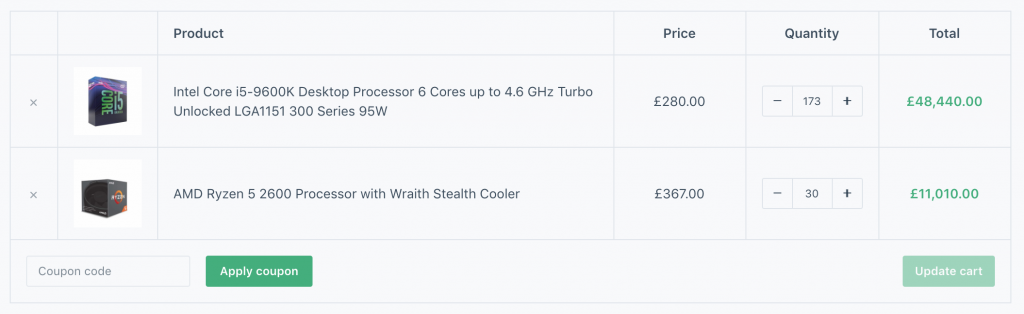In this image, a detailed view of an online shopping cart is displayed. The cart contains two prominently listed items, likely components for computer systems.

1. **Intel Core i5-9600K Desktop Processor:**
   - **Specifications:** 6 cores, turbo speed up to 4.6 GHz, unlocked, LGA1151-300 series, 95 watts.
   - **Price:** £280
   - **Quantity:** 173 units
   - **Total Cost:** £48,440

2. **AMD Ryzen 5 2600 Processor with Wraith Stealth Cooler:**
   - **Specifications not detailed in text.**
   - **Price:** £367
   - **Quantity:** 30 units
   - **Total Cost:** £11,010

Below these listings, there is a green button labeled for applying coupon codes and a grayed-out "Update Cart" button. The total value of the cart exceeds £55,000, indicating a substantial purchase.

The cart, designed with a simple, gray rectangular box, includes clearly separated sections for product details, price, quantity, and total amount, suggesting it is part of an e-commerce website’s interface.